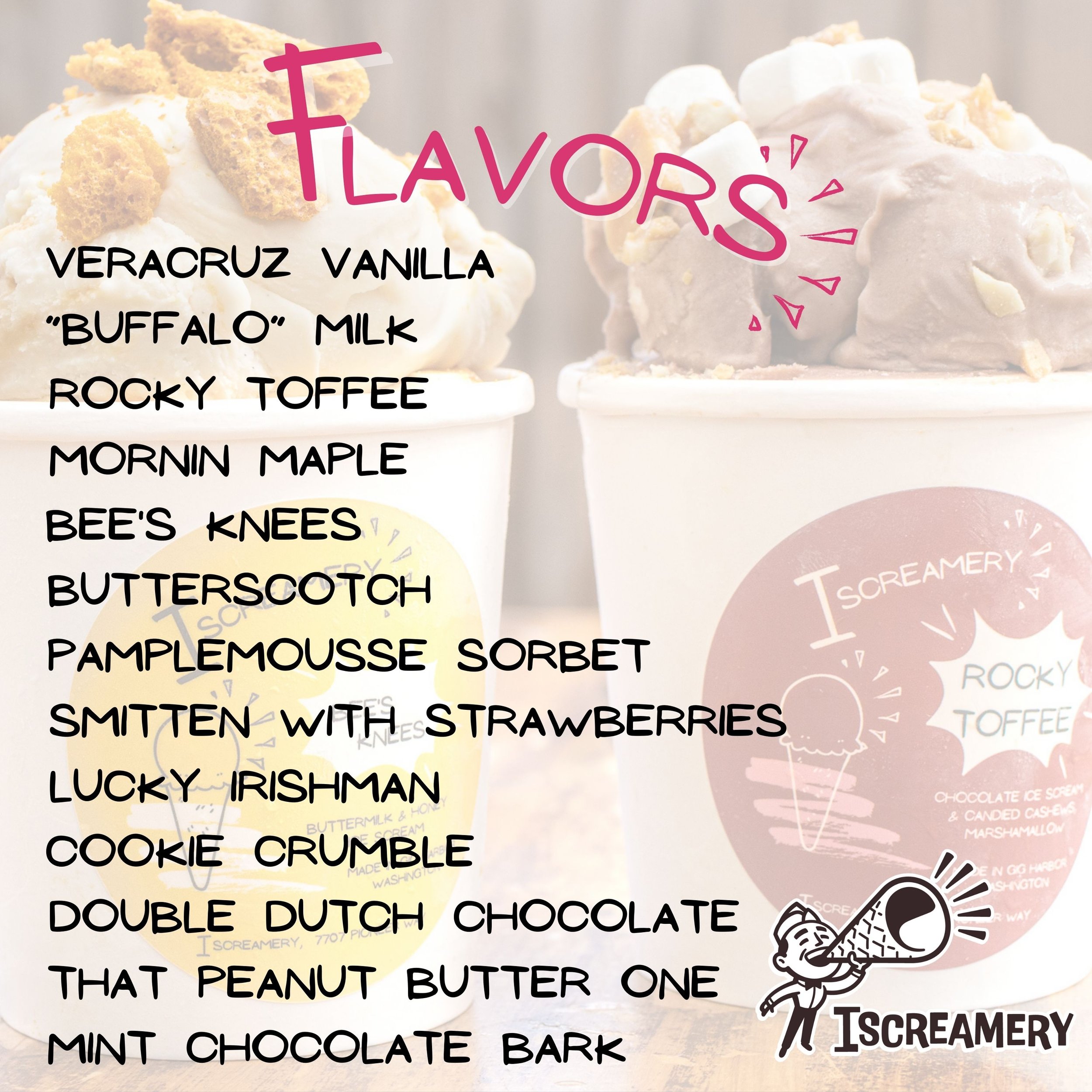This is a colorful and playful advertisement poster for iScreamery, a high-end creamery offering unique ice cream flavors. The top of the poster features the word "Flavors" in a fun pink font, superimposed over a background image of two cups of chunky, delicious-looking ice cream. Listed in black text are enticing flavors including Vera Cruz Vanilla, Buffalo Milk, Rocky Toffee, Morning Maple, Bees Knees Butterscotch, Pamplemousse Sorbet, Smitten with Strawberries, Lucky Irishman, Cookie Crumble, Double Dutch Chocolate, That Peanut Butter One, and Mint Chocolate Bark. At the bottom right corner, the iScreamery logo showcases a character wearing a traditional restaurant hat, shouting through an ice cream cone megaphone, cleverly playing on the words “I scream” and “creamery.” The overall design is vibrant and tempting, promising a delightful array of ice cream options.